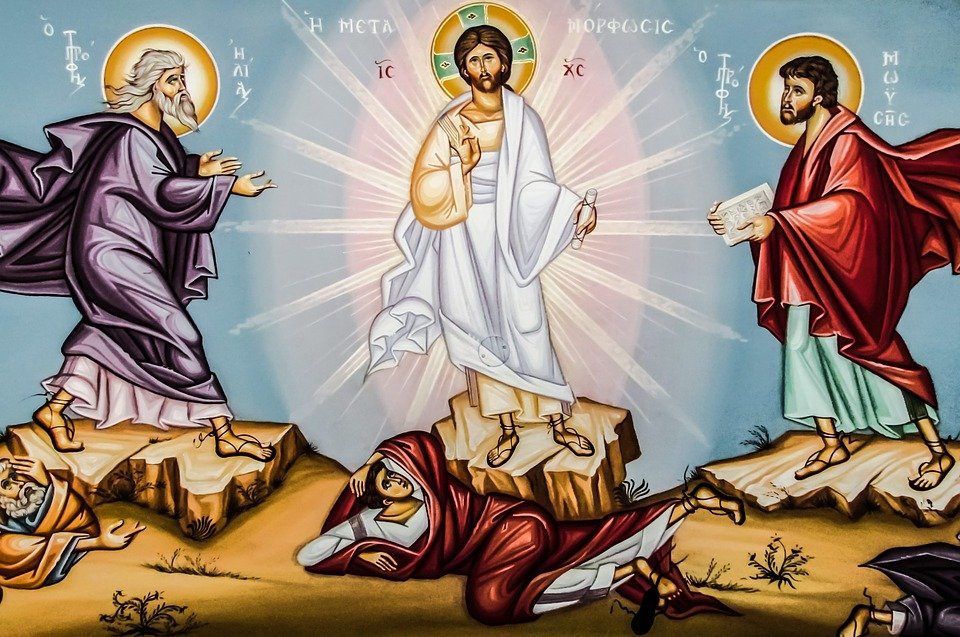This illustration vividly depicts a religious scene featuring four figures with a strong focus on a central figure, likely representing Jesus Christ. The central figure, dressed in a golden and white robe with sandals, has long brown hair, a beard, and rays of light emanating from behind him, forming a halo. He stands authoritatively above a man lying on the ground, who is covered in a red outfit and gazes up at him with a look of reverence. On the left of this central figure stands an elderly man with long white-grey hair and a matching beard, draped in a purple robe, extending his hands towards the central figure. On the right, another bearded man in a red cloak with white underneath stands, also looking towards the central figure. Additional details in the image include Greek letters and words such as "H. Meta," "IC," and "XC," contributing to the deeply historical and religious atmosphere. The scene is bathed in sunlight that enhances the divine aspect of the tableau.